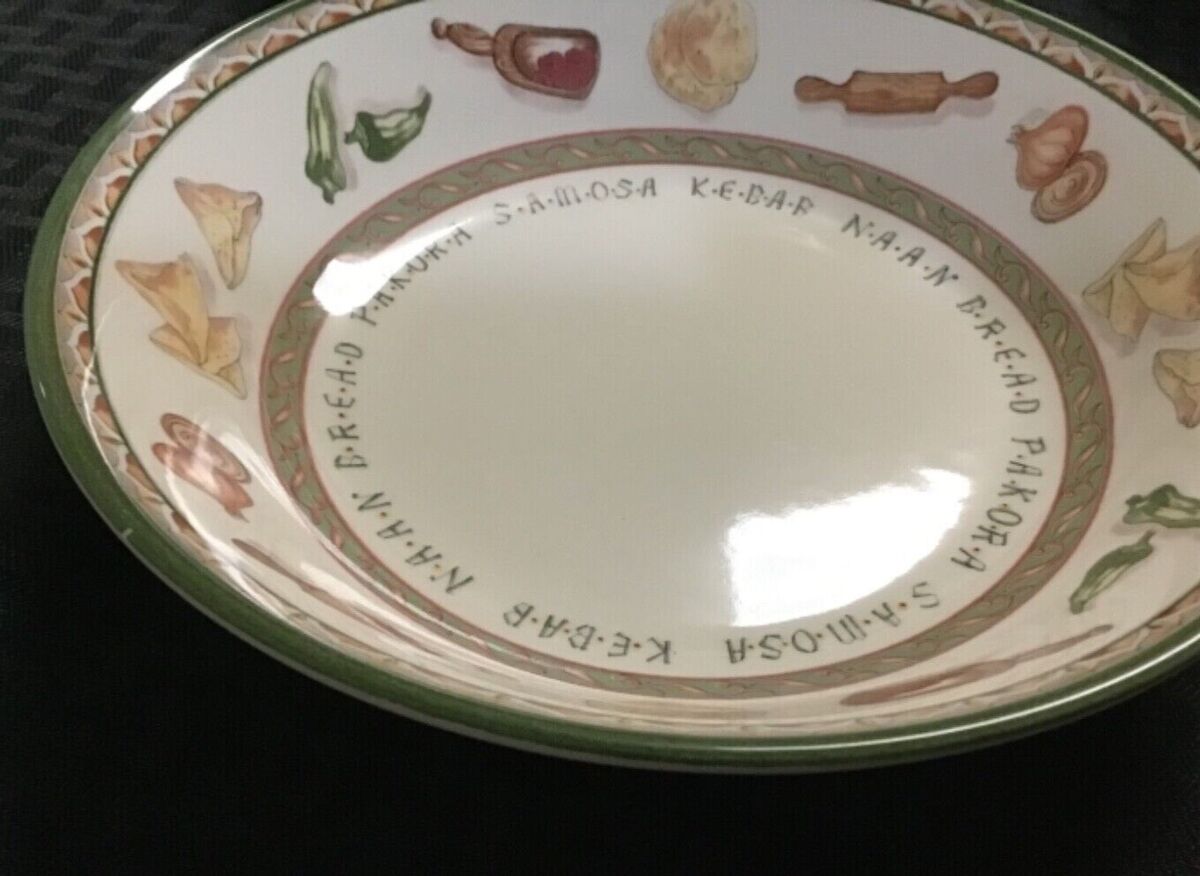This image, taken in landscape orientation, features a wide, bowl-shaped ceramic serving dish placed on a grey and black patterned surface. The dish has a prominent olive green lip, followed by an intricate floral or petal design along the inner edge. Below this design are colorful illustrations of various vegetables and kitchen items, including okra, onions, peppers, and a wooden rolling pin, arranged around the interior perimeter. The base of the bowl is white with multiple instances of the words "naan, bread, pakora, samosa, kebab" written in a circular pattern. Reflections of light are visible on the polished surface of the bowl, enhancing the detailed and vibrant imagery throughout. The bottom half of the image shows a peach-black color, offering a stark contrast to the more intricate elements of the bowl's design.